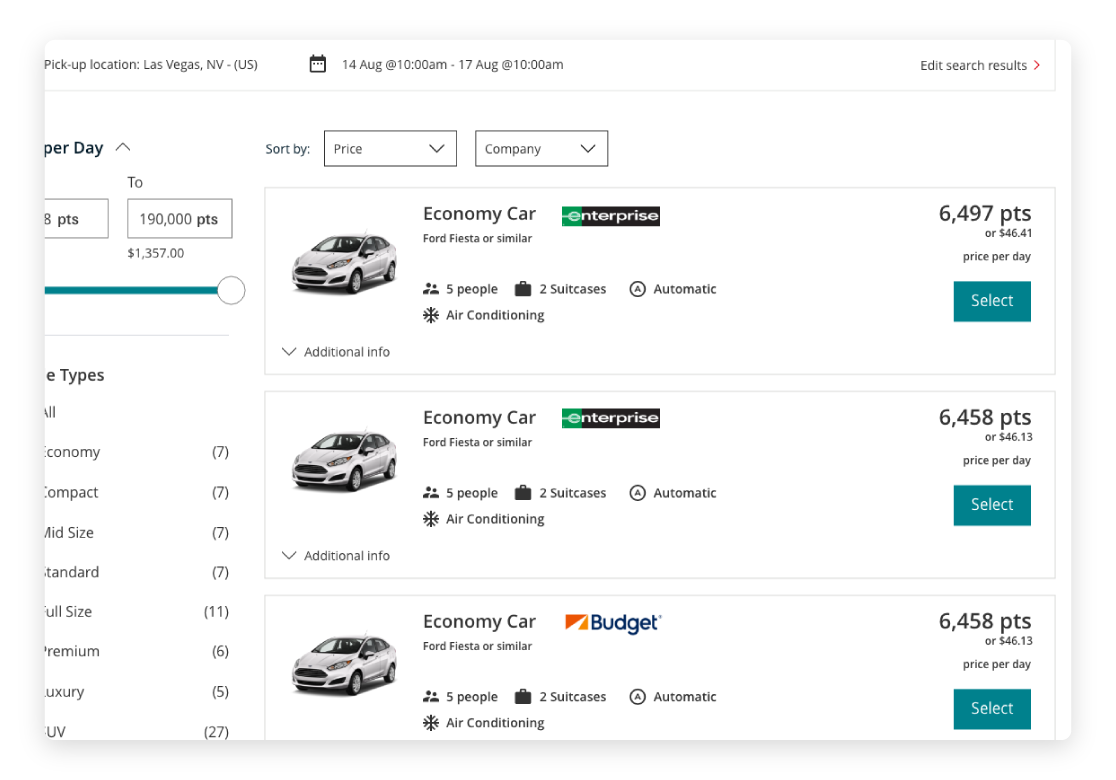The image displays a clean, white-background website interface for booking rental cars. In the top left corner, it reads "Pick-up Location: Las Vegas, Nevada (US)." Below this, a calendar indicates the rental period from 14 August at 10 a.m. to 17 August at 10 a.m. To the right, there is an option to "Edit Search Results," highlighted by a red right arrow.

Descending the page, a partially visible section shows rates "PER day" with an up arrow. There are two fields indicated by rectangles; one specifies "APTS" with a cost of "190,000 points," while the other shows "$1,357."

Further down, a horizontal banner details car types, including economy, compact, mid-size, standard, full-size, premium, luxury, and SUV. This section is somewhat cut-off vertically. Adjacent to this, the site offers sorting options "by Price" and "Company," accessible via a drop-down menu.

The lower part of the image showcases three rental car options: each listed as an "Economy Car, Ford Fiesta or similar" from agencies like Enterprise and Budget. On the right side of each car listing, the pricing is shown in points or dollars per day.